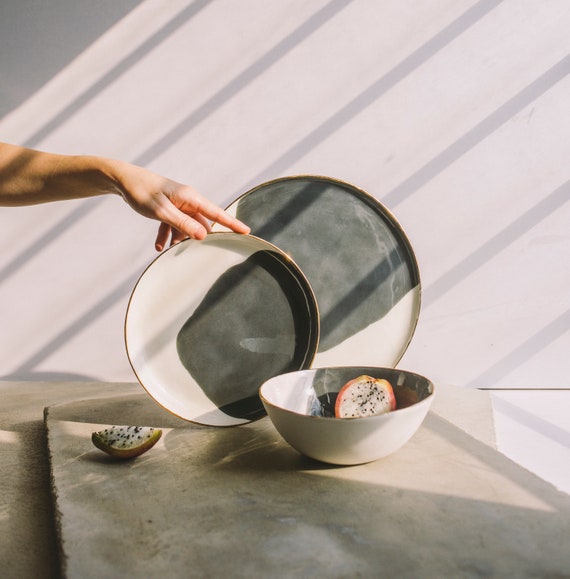The professionally taken, square-shaped photograph captures a serene still-life scene in a well-lit room. The background features a white wall adorned with shadowy, striped patterns likely formed by sunlight streaming through a window. At the center of the image is a substantial concrete table. An adult's left hand, characterized by white skin, reaches into the frame from the right side, holding a medium-sized ceramic plate with a distinctive design—white with a large black splotch and a gold rim. Behind this plate, a larger plate bearing the same pattern is visible. Also on the table is a matching bowl, inside which lies half of a fruit that could be an apple speckled with black seeds or perhaps a kiwi. Another slice of the fruit rests on the table beside the bowl.